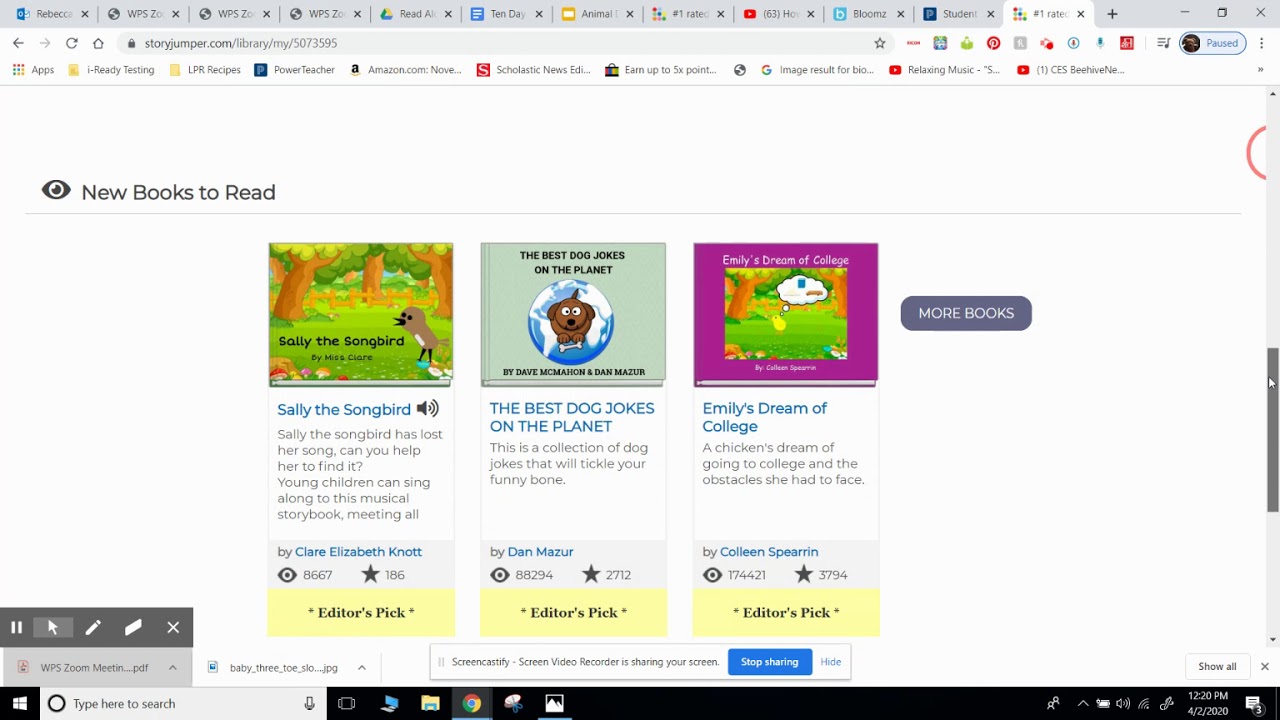A screenshot capturing a busy digital workspace. The desktop features a Chrome browser with several open tabs. Visible icons include 'Data Search,' 'Folder,' and 'Snip & Sketch.' The system tray displays a fully charged battery and the current time, 12:20 PM, on April 2, 2020.

In the browser, multiple tabs can be discerned, labeling various projects and interests: 
1. "Pop Flash - says Rebecca."
2. "WPS, WPS3, Dente, Animal,"
3. File number "180, 6310,"
4. "YouTube" 
5. "Bloom Studio."

A specific tab highlights "storyjumper.com/library/my/5073591," featuring a children's musical storybook titled "Sally the Sombrero's Lost Song" by Claire Elizabeth Knot. The narrative invites young readers to help Sally find her lost song, encouraging sing-alongs and interactive engagement.

Bookmarks include diverse entries like "Testing," "LPR Recipes," "PowerTeacher," "Amazon.com Classic," "News," "Winter Adult," "Books and Music," and "CSBI Use Books to Read."

Aligned bookmarks are:
- "Star icons 123456789"
- "Best Dog Jokes on the Planet," a collection of humorous dog jokes
- "Emily's Dream of College," a pursuit for college education
- "My Chicken and His Dream of College Without a Scholarship," a whimsical story about a chicken aspiring for higher education.